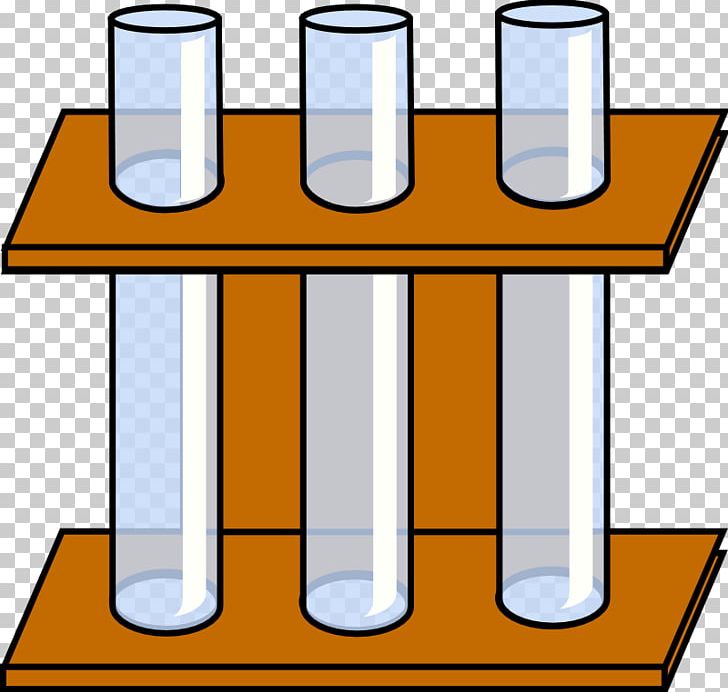This image is a detailed digital illustration of three clear, glossy test tubes with a light blue tint, perfectly centered and taking up most of the screen. Each test tube is held upright in a brown holder, which appears to be made of wood, featuring two horizontal panels that keep the tubes steady. The top panel has three holes while the bottom has three notches, ensuring the test tubes remain vertical. The entire background of the image is a white and gray checkered pattern, indicating that the final design is intended to have a transparent background. The illustration is in a clip art style, likely for online use, and there is no text visible within the image.